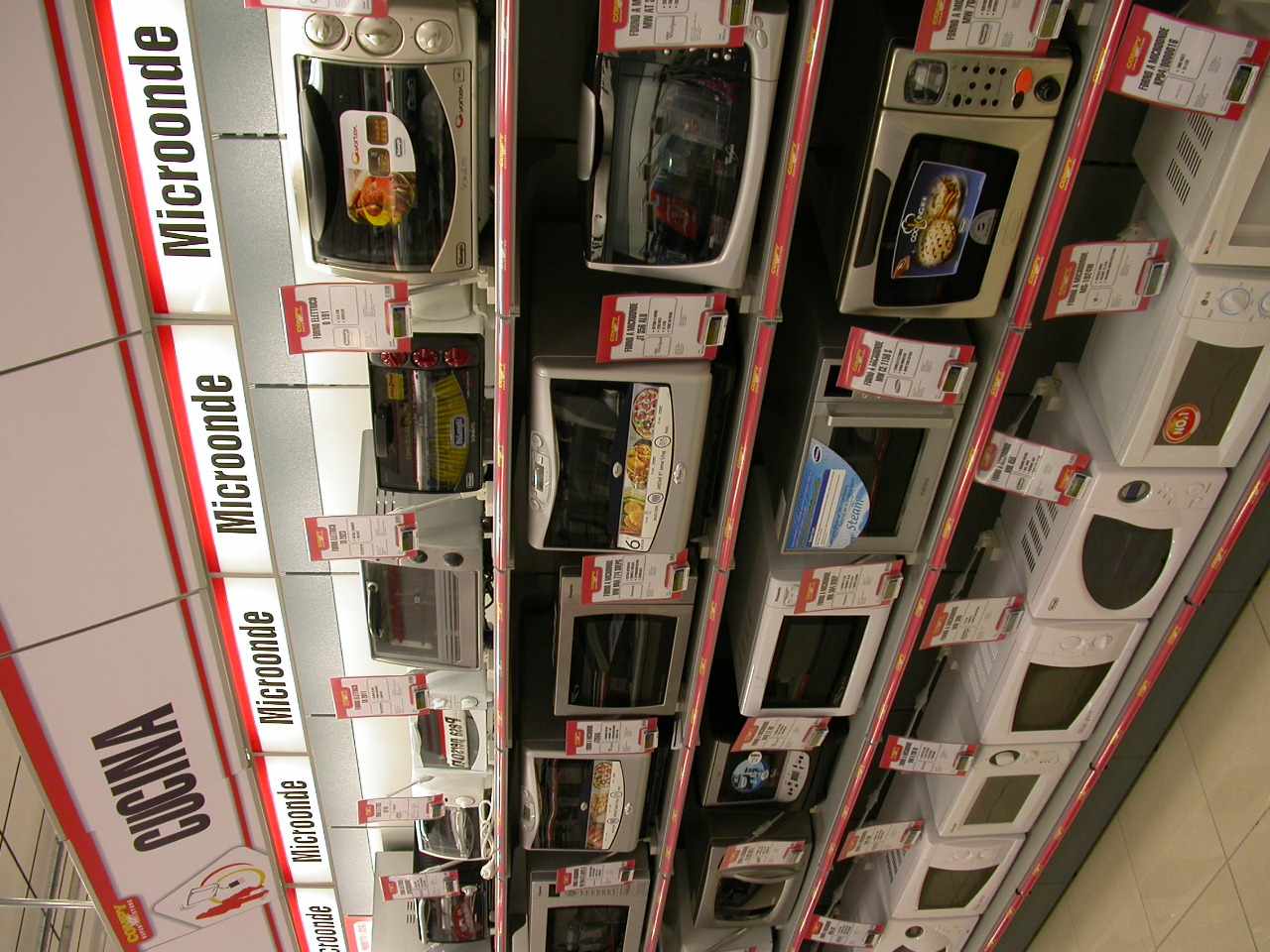This image, oriented sideways, depicts a department store display of various cooking appliances, primarily microwaves, across several shelves. The floor, partially visible, consists of large cream porcelain tiles. On the bottom shelf, starting from the bottom left corner, there is a white shelf with a gray front edge, and a notable red and white tubing draped in front. This shelf holds different models of white microwaves with black fronts that appear unlit.

Moving up, the next shelf has a similar setup with a gray top and a red border featuring yellow lettering. From the right, the lineup includes two silver microwaves, a white microwave, a black microwave, and another silver microwave, followed by yet another row-like border with red and yellow writing. Continuing leftward, this shelf displays a short silver microwave, a large boxy silver microwave, a standard-looking microwave, another similar large silver microwave, and finally, a silver microwave.

The topmost shelf showcases a variety of appliances, beginning from the right: a large square silver microwave, a black microwave with three prominent red buttons on the right side, a silver toaster oven farther back, two small white microwaves, and a small black microwave on the far left. Above the appliances, a white border with black lettering spells out "MICRON DAY," and above that, a large white sign with "CUCINA" in black text and a red border on top and bottom.

The overall display is brightly lit, with shelf tags presumably listing features and prices for each appliance. To properly view the image as described, it should be rotated counterclockwise so that the top of the picture aligns correctly on the left side.